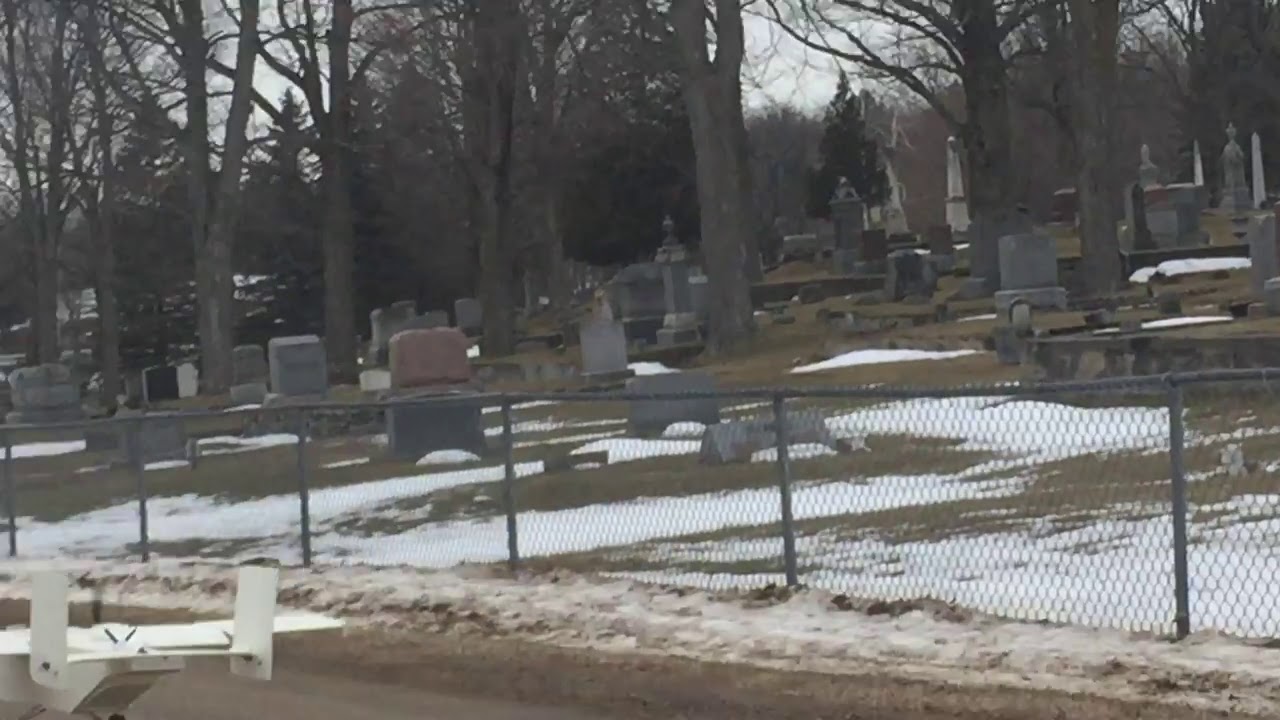Set against a gray, overcast sky, this winter cemetery scene is both serene and somber. The ground is partially covered in patches of muddy, dirty snow, revealing tufts of green grass beneath. Enclosing the cemetery is a silver or gray chain-link fence, partially obscured by small banks of snow. The graveyard is dotted with an array of tombstones and gravestones in varying shades of gray and brown, including taller, pillar-like stones and even a few obelisk-shaped monuments in the distance. Surrounding the tombstones, leafless deciduous trees with gray trunks stand tall, interspersed with triangular-shaped coniferous trees that retain their dark green needles. In the background, large towering tree trunks add to the scene's stark winter atmosphere. Notably, on the far left-hand corner of the image, the white tail of a vehicle or drone peaks from the frame, adding a subtle modern touch to this timeless setting.